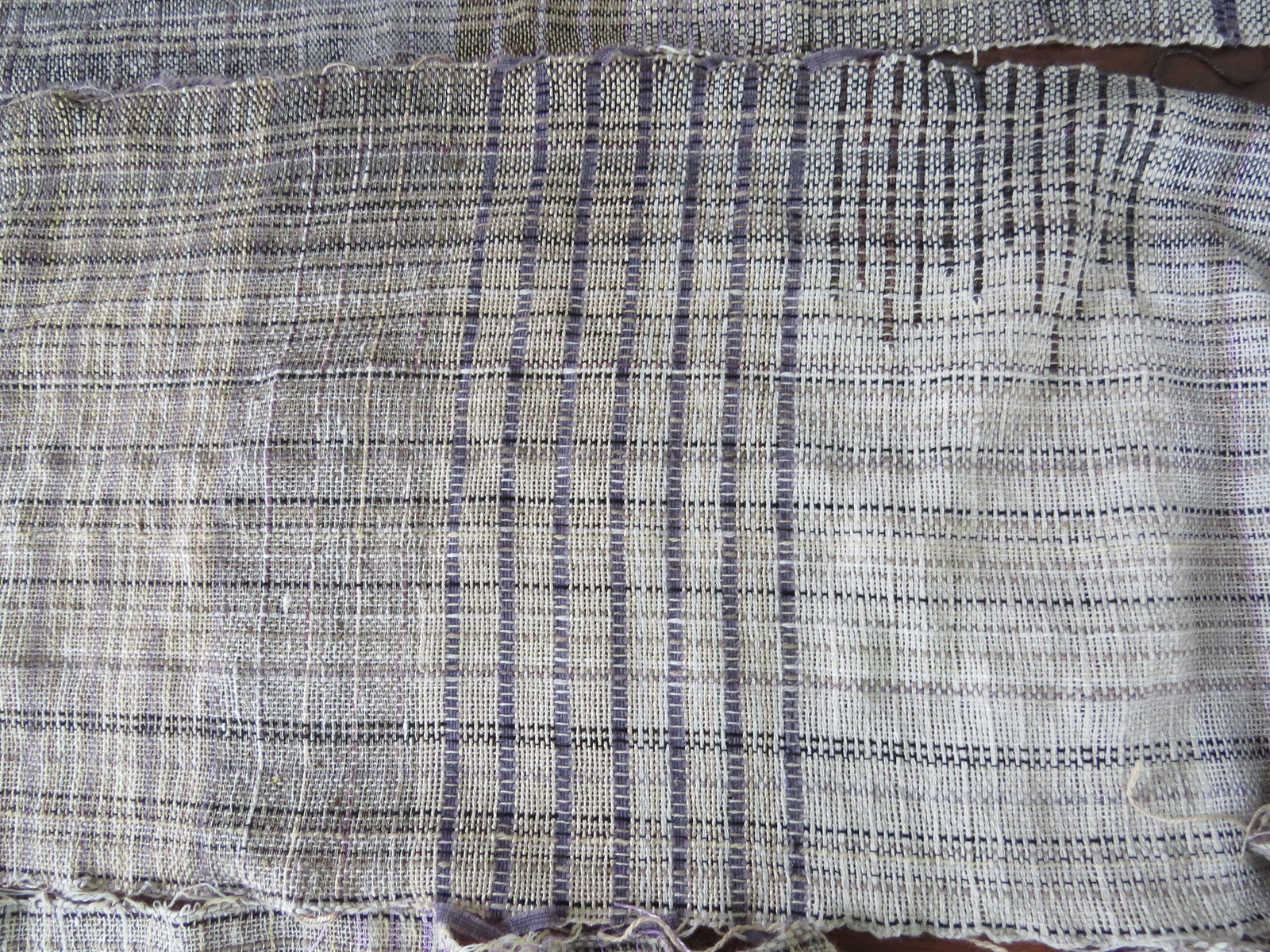This close-up image showcases a piece of fabric, potentially a tablecloth or placemat, that appears worn with some frayed edges and loose threads. The fabric exhibits a rough texture and comes in a multicolor palette of tan, light blue, off-white, and gray, with a visible sliver of a brown table peeking between it and another similar piece of fabric. The main fabric displays a pattern of seven vertical blue stripes, complemented by several horizontal dotted lines in blue and black, imparting a patchwork or plaid appearance. Additionally, there are indications of black and dark blue stripes alongside yellow stitching which may be part of its decorative design. In the background, another piece of fabric from the same set is visible, featuring a similar color scheme but with gold stripes. The overall composition reveals a richly patterned and perhaps vintage fabric set.